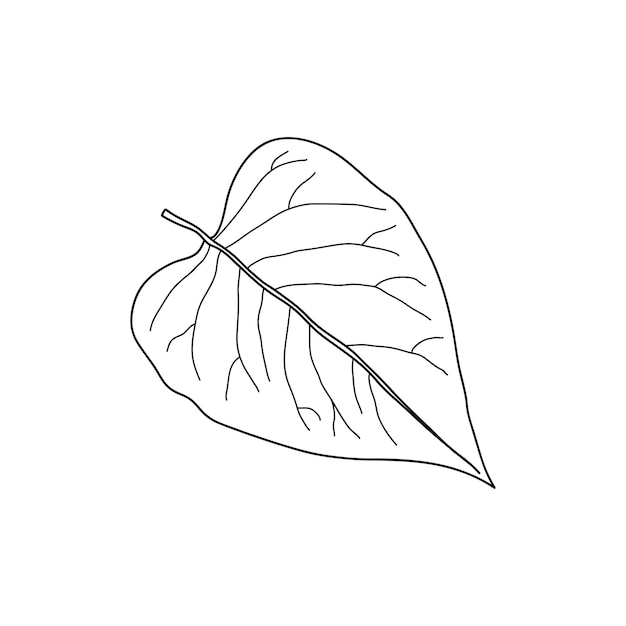The image depicts a hand-drawn or computer-generated, black-and-white ink illustration of a single leaf. The leaf is simplistic yet richly detailed, showcasing its central rib from which veins extend outward. It features a heart-shaped design with a prominent V-like notch at the top. The stem runs down the center, branching out into five veins on the upper section and eight veins on the lower section. The detailed veins are designed to represent the leaf’s role in photosynthesis, highlighting how it distributes nutrients essential for plant growth. Its clear and minimalistic style makes it suitable for educational purposes, such as coloring activities or diagrammatic presentations, and evocative of a leaf in different seasonal cycles like spring and fall.